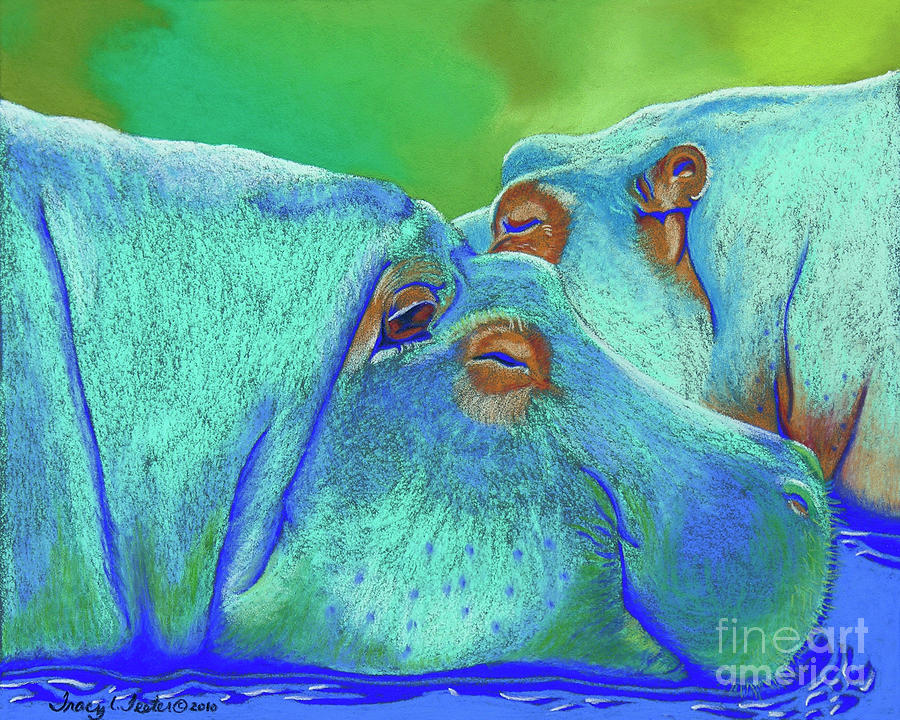This vibrant digital painting by Tracy Tester, copyrighted in 2010, features two hippopotamuses partially submerged in a pond. The dominant hippo in the foreground takes up most of the image, with its head fully visible and only a hint of its body to the left. The second hippo, positioned behind it, is partially obscured; only its closed eye, ear, and part of its body are visible, as its mouth is blocked by the front hippo. The water is vividly depicted with varying shades of blue and green, accentuated by ripples at the bottom, suggesting the hippos are submerged. The hippos themselves are mainly blue with greenish hues around their noses and mouths, and they have brownish highlights around their eyes and ears. The background transitions to a lush green with darker green and brown elements resembling grass or trees. The image has a text overlay at the bottom right corner that reads "Fine Art America" in white, and the artist's name, Tracy Tester, along with a copyright symbol and the year 2010, is placed prominently. The overall scene suggests a peaceful moment with the hippos either napping or relaxing in the water under a bright, vibrant background.